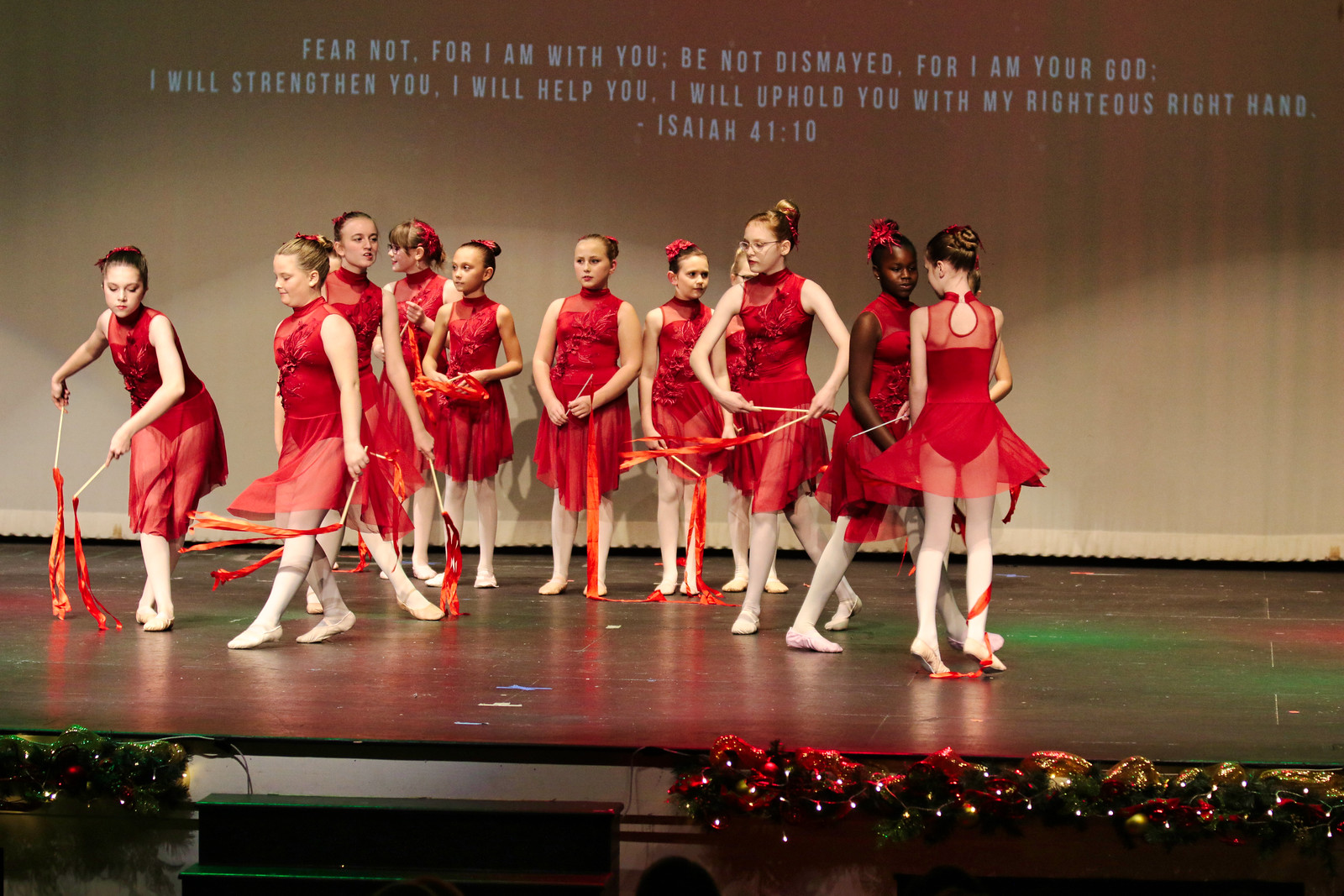The photograph depicts an indoor stage with a dozen pre-teen to young teen girls, likely between the ages of 10 and 14, dressed in sleeveless red ballet dresses accompanied by sheer red skirts, white tights, and ballet slippers. Each girl holds sticks adorned with red and yellow ribbons. They have their hair styled in braids and appear to be either practicing or preparing for a dance performance. The stage has a dark brown wooden surface, accented by green and multi-colored stage lighting. In the background, a scripture from Isaiah 41:10 is projected in all capital letters: "FEAR NOT, FOR I AM WITH YOU; BE NOT DISMAYED, FOR I AM YOUR GOD; I WILL STRENGTHEN YOU; I WILL HELP YOU; I WILL UPHOLD YOU WITH MY RIGHTEOUS RIGHT HAND." The backdrop is a pale, tan-colored curtain. The edge of the stage is decorated with holiday garland and Christmas lights, hinting at a festive season. At the bottom of the photograph, two green steps lead up to the stage. The audience is partially visible, with the backs of some spectators' heads in view.